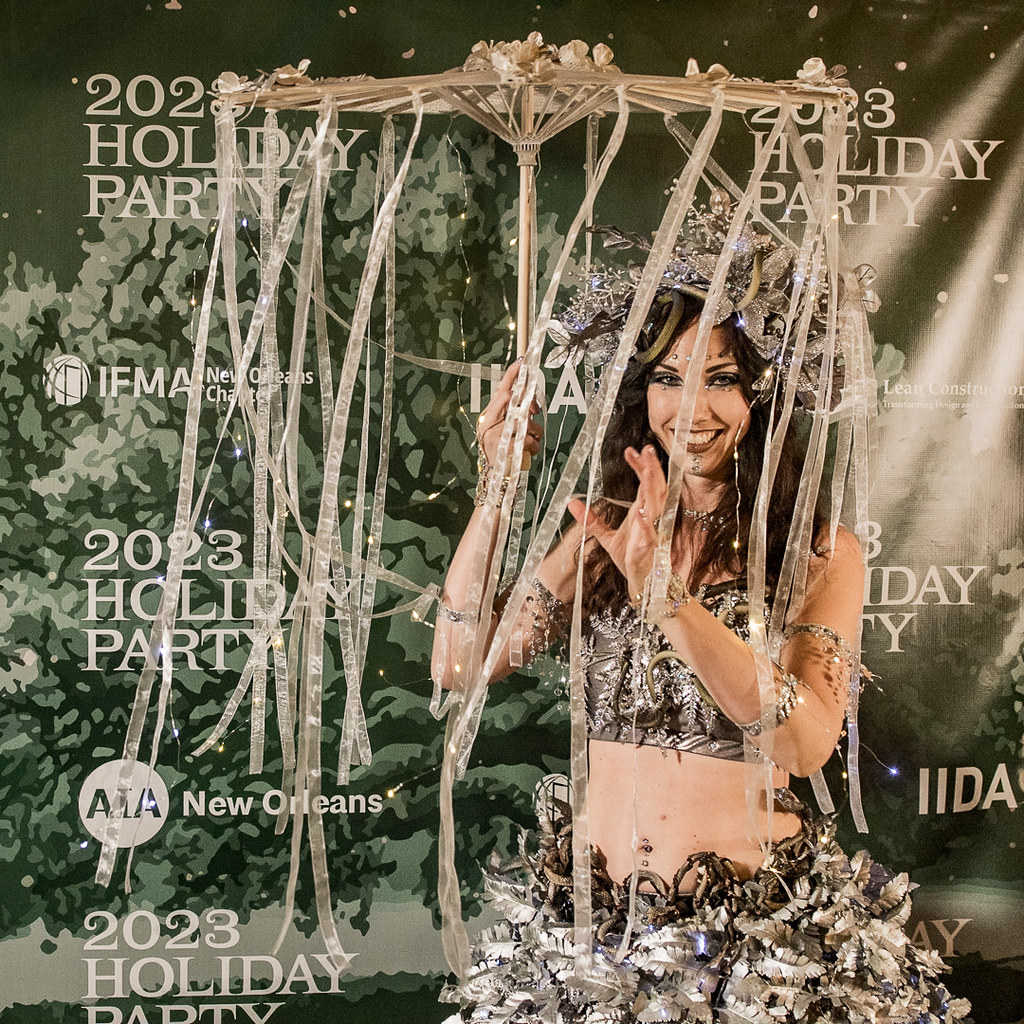The image depicts a woman at a bustling 2023 Holiday Party hosted by the IFMA New Orleans Chapter. She's wearing an elaborate, sculptural outfit that appears to be made of curled materials resembling either pop cans or metallic leaves, creating a striking, shiny texture reminiscent of ornamental Christmas tree decorations or silver tinsel. The outfit includes a crop top, revealing her pierced belly button, and a matching headdress that encircles her head. She holds a large decorative parasol, which looks like a capital T fashioned from bamboo, adorned with cascading white streamers. The woman stands in front of a stylized painting featuring tree motifs and the event's name. Smiling, she reaches up with one hand as if to brush back the streamers, adding to the festive and dynamic atmosphere captured in the photograph.